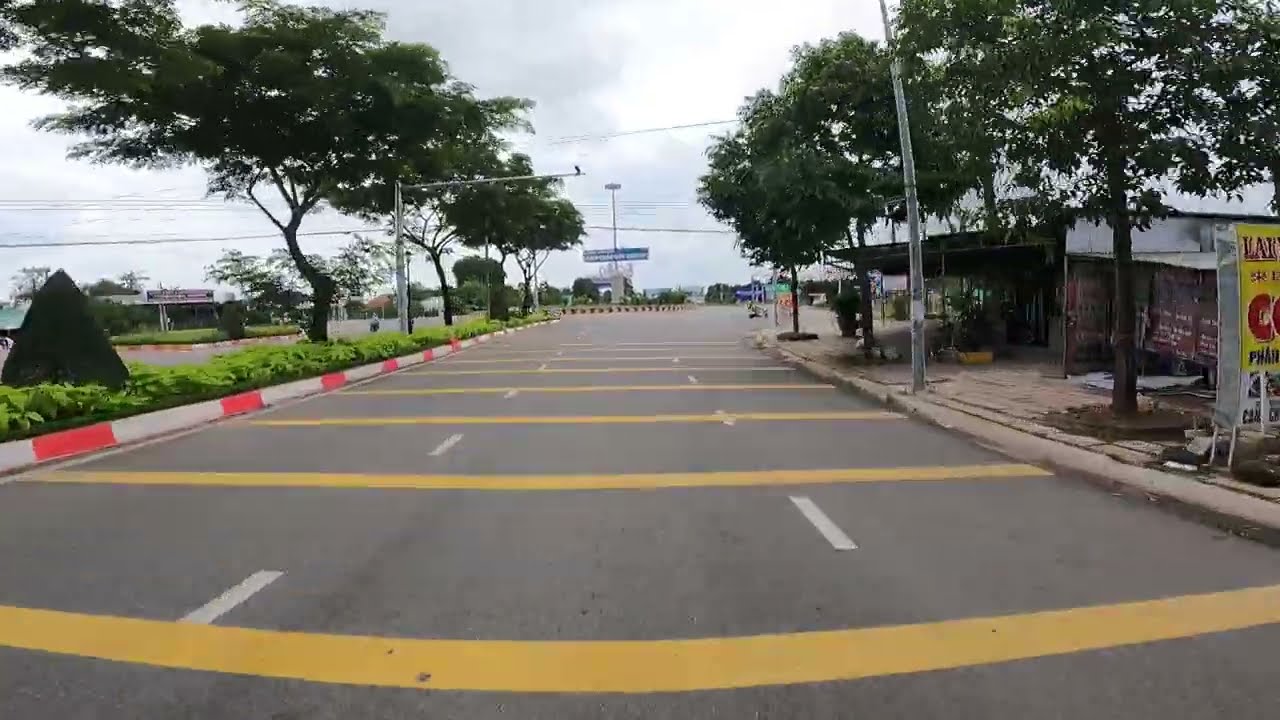The daytime image captures a potentially foreign, wide, three-lane road bordered by tall pine trees and characterized by unique markings. The road is patterned with yellow horizontal lines resembling raceway stripes and dotted vertical white lines evenly spaced to delineate the lanes. A median in the middle left of the image features a grassy area with a distinct cone-shaped tree, divided by red and white patterned curbs. The left and right edges of the road also bear this candy-cane stripe pattern. In the background, power lines stretch across the scene, contributing to the urban yet natural ambiance. A clean sidewalk runs along the side of the road, where a billboard and small shacks or street vendor-like structures are visible. The sky, partly cloudy with blue patches, suggests a bright yet overcast day, devoid of any vehicles or pedestrians. A shelter-roofed building stands on the right, reinforcing the scene's potential location in a foreign downtown area.